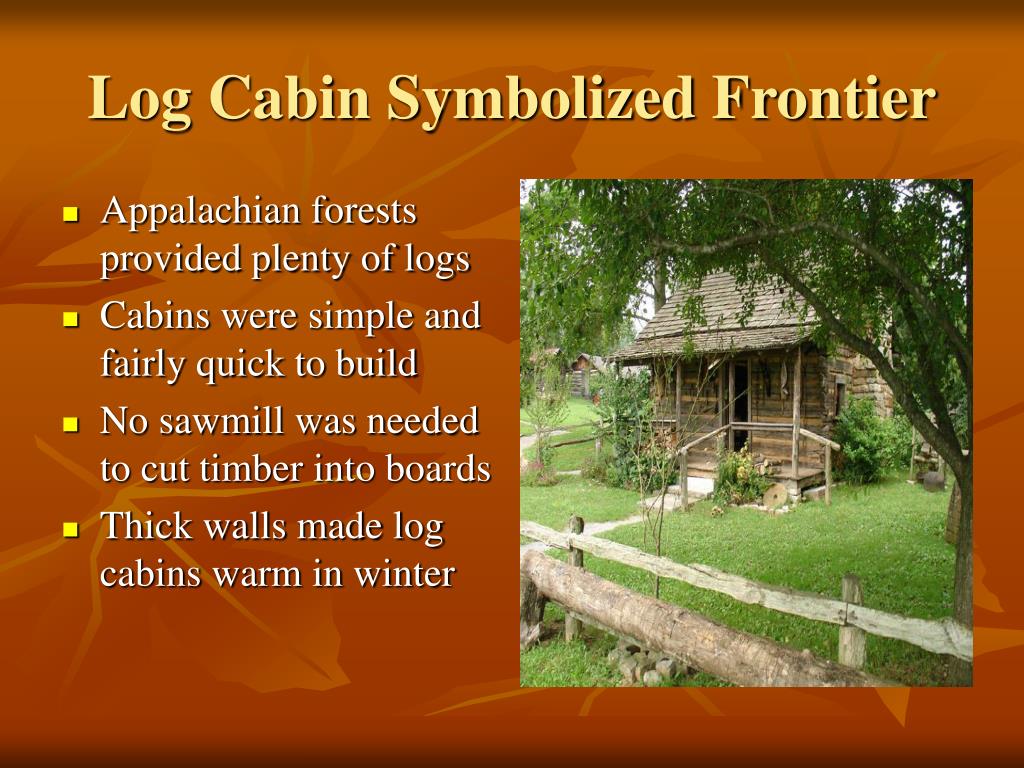The image, titled "Log Cabin Symbolized Frontier" in yellow Times New Roman font at the top, features a detailed depiction of a small log cabin surrounded by lush greenery. Positioned to the right, the cabin stands on vibrant green grass with a simple wooden rail fence enclosing the front yard. A large green tree adorns the yard, its branches extending over the cabin. The cabin itself is basic, featuring a door, a simple porch, and one visible front window, with a short walkway leading up to it. To the left of the cabin picture, there are four yellow square bullet points with white text that highlight the key aspects: "Appalachian forests provided plenty of logs," "Cabins were simple and fairly quick to build," "No sawmill was needed to cut timber into boards," and "Thick walls made log cabins warm in the winter." The background of the entire image is a dark rusty orange with a print of sketched, clip-art style leaves, creating a rustic atmosphere.